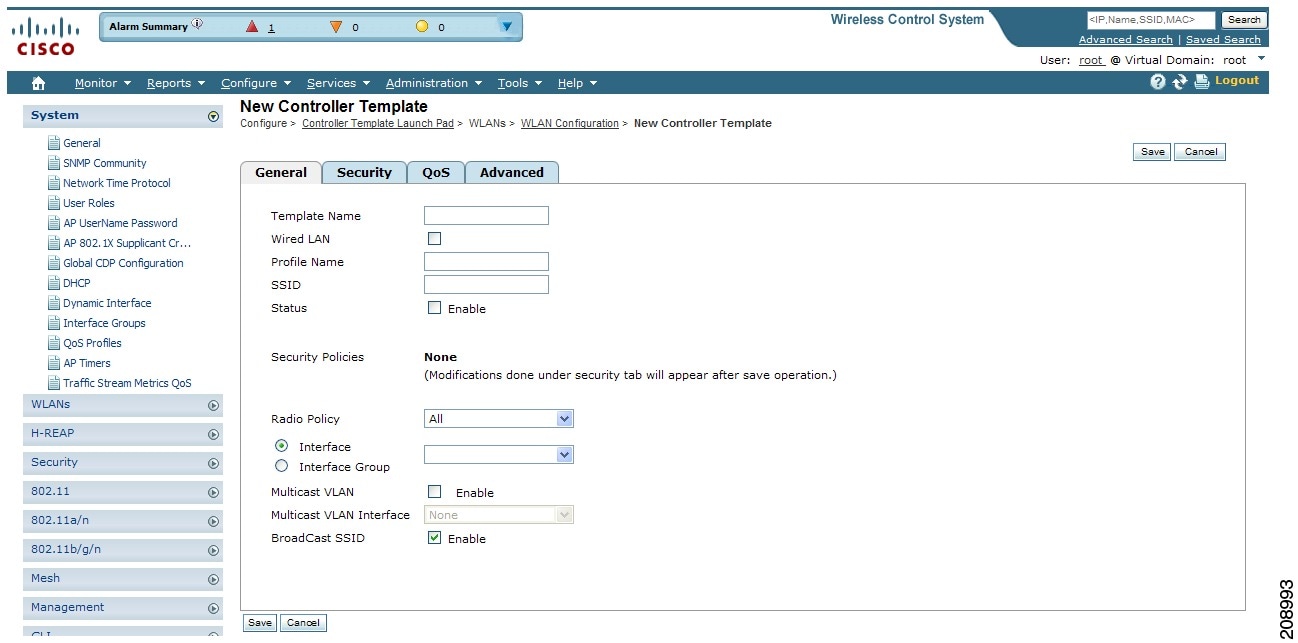**Detailed Caption:**

The image depicts the login screen for Cisco's wireless control system panel. At the top, there's an alarm summary section with various icons: a red triangle with a number '1' indicating an alert, an orange downward-facing triangle with a '0', and a yellow circle with a '0'. On the upper right-hand corner, there are login fields for user authentication. 

Below this, a blue navigation bar houses several options, including "Monitor," "Reports," "Configure Services," "Administration Tools," among others. On the left side, there is a collapsible menu containing an array of options such as WLANs, H-REAP, Security, 802.11 settings, Mesh, and Management.

The screen currently displays the "New Controller Template" creation view. Within the general tab, there are numerous customizable settings comprising template name, wired LAN, profile name, SSID, status, security policies, radio policy, multicast VLAN, and broadcast SSID. At the bottom of the page, two buttons allow the user to save or cancel the configurations. The layout is structured to facilitate the creation and management of a wireless controller template efficiently.